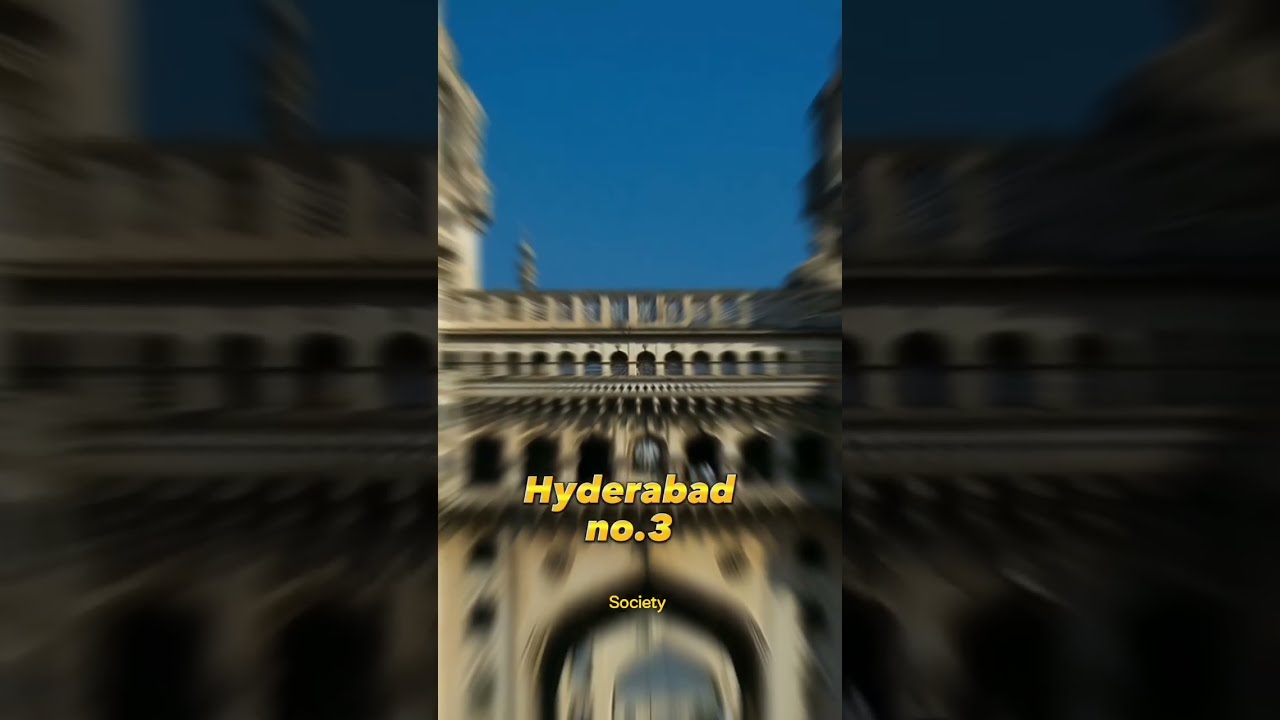This photograph, captured in portrait mode using a cell phone, prominently features a grand stone arched building, exuding an architectural style reminiscent of the Italian Renaissance. Dominating the center of the image, the facade reveals a meticulously detailed structure composed of multiple archways and windows. At the base, a large entryway arch leads through to an unseen internal space, while directly above it is a colonnade of smaller arches, topped by a row of similarly arched windows. Further up, the building is adorned with a sequence of square windows. The backdrop of the photograph is a clear, vivid blue sky, with partially visible towers framing the scene to the left and right, adding to the building’s majestic appearance.

The image appears to have a motion blur effect, creating the sensation of rapidly approaching the building, further emphasizing its grandeur and giving it a dynamic and almost surreal ambiance. The entire composition is overlaid with bold, golden text that reads "Hyderabad No. 3" with a subtext below stating "society" in the same golden hue. These textual elements float prominently over the image, adding a modern, almost ethereal contrast to the historic architectural beauty depicted in the photograph.